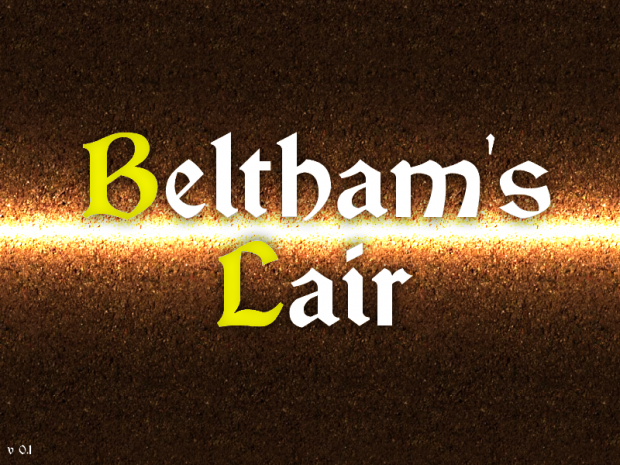The image depicts a splash screen of a game titled "Beltham's Lair." The title is rendered in a medieval-style font, with "BELTHAM" at the top and "LAIR" at the bottom. The initial letters "B" and "L" are highlighted in yellow, while the other letters are in white. The background of the image features a horizontal, gold-yellow glowing stripe that illuminates the center, transitioning from dark brown at the top and bottom to a lighter golden brown towards the center. The texture appears gritty and has a metallic look. In the bottom left corner, the small text "V 0.1" indicates the version number, suggesting this is an early version of the game.